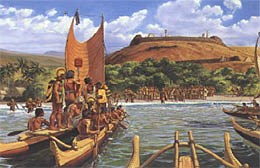In this small, detailed image, several double-hulled Polynesian outrigger canoes with sails are depicted heading toward shore. The canoes, loaded and brown in color, are manned by dark-skinned people with dark hair, wearing loincloth-like attire. Some boats appear somewhat overloaded, while others show just the bow or appear empty. The people onboard are rowing, and more people can be seen on shore, seemingly awaiting their arrival. The image is set against a backdrop of rich blue skies with fluffy white clouds. The green island features a prominent hill topped with a dug-out structure, possibly a temple or arena. The hill is mostly dirt, adorned with trees at its base. The scene encapsulates a vivid moment of indigenous life, highlighting their sophisticated watercraft and communal interaction.